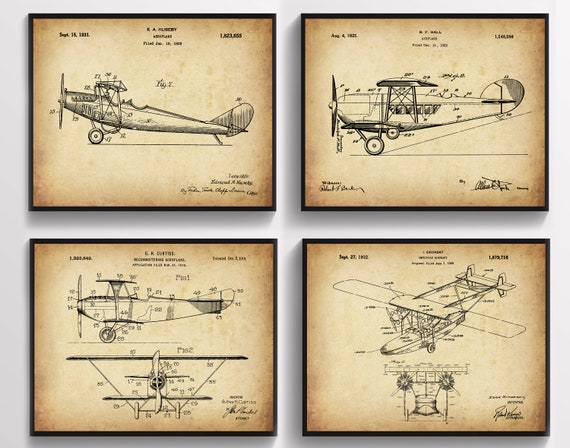This product image showcases a set of four framed posters, meticulously presented against a featureless white wall in the simplistic style common in commercial photography for online shops or catalogs. Each poster is enclosed in a thin black rectangular frame and printed on a tan, parchment-like paper that darkens towards the edges. The posters are arranged in a grid—two on the top and two on the bottom—and display detailed black ink schematics of early 1900s propeller-driven airplanes.

The top left poster features a side view of a plane with lines of text surrounding it, including a date, "September 13, 1919," in the top left corner. The other posters similarly showcase planes with black and white line drawings, complete with labels and arrows pointing to different parts of the aircraft. The bottom right image notably depicts a seaplane or float plane. Each schematic is meticulously detailed, with two of the bottom images showing planes from different perspectives: one from the front and the other from an angled viewpoint. The minimalistic gray shading effect accentuates the background, ensuring the vintage aesthetic of the framed drawings remains the focal point.